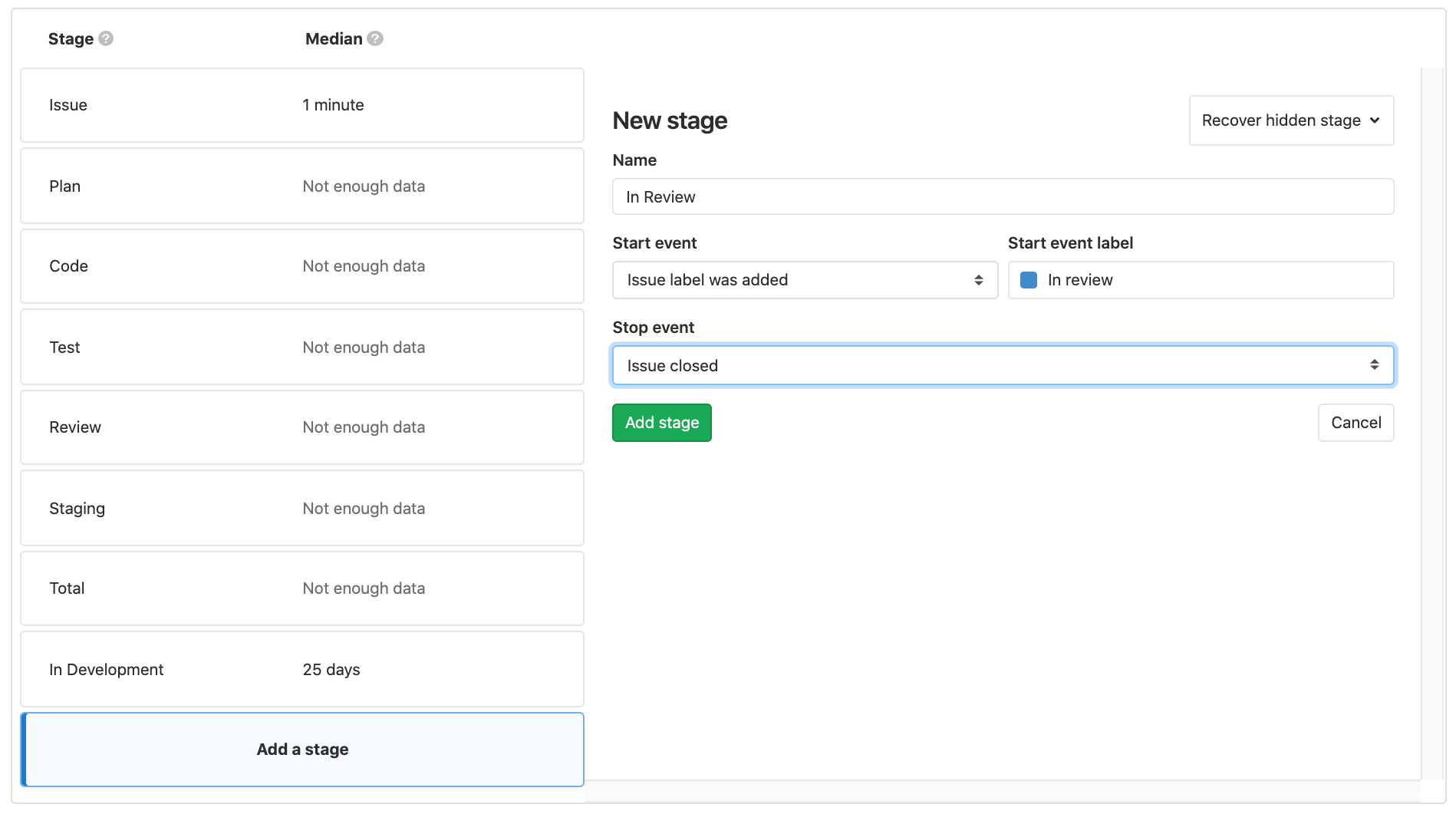This image depicts a web page likely used for event planning or project management, focusing on scheduling and organizing various stages of a project. At the top left corner, the page features the label "Stage," and directly to the right is a label reading "Median." Below "Stage," there are several listed options including "Issue," "Plan," "Code," "Test," "Review," "Staging," and "Total." The final stage, "In Development," is indicated with a timeline of "25 days." Just underneath, there's a prominent blue-highlighted rectangular button labeled "Add a Stage." In the center of the page, a green "Add Stage" button is prominently displayed, alongside a "Cancel" button positioned to its right.